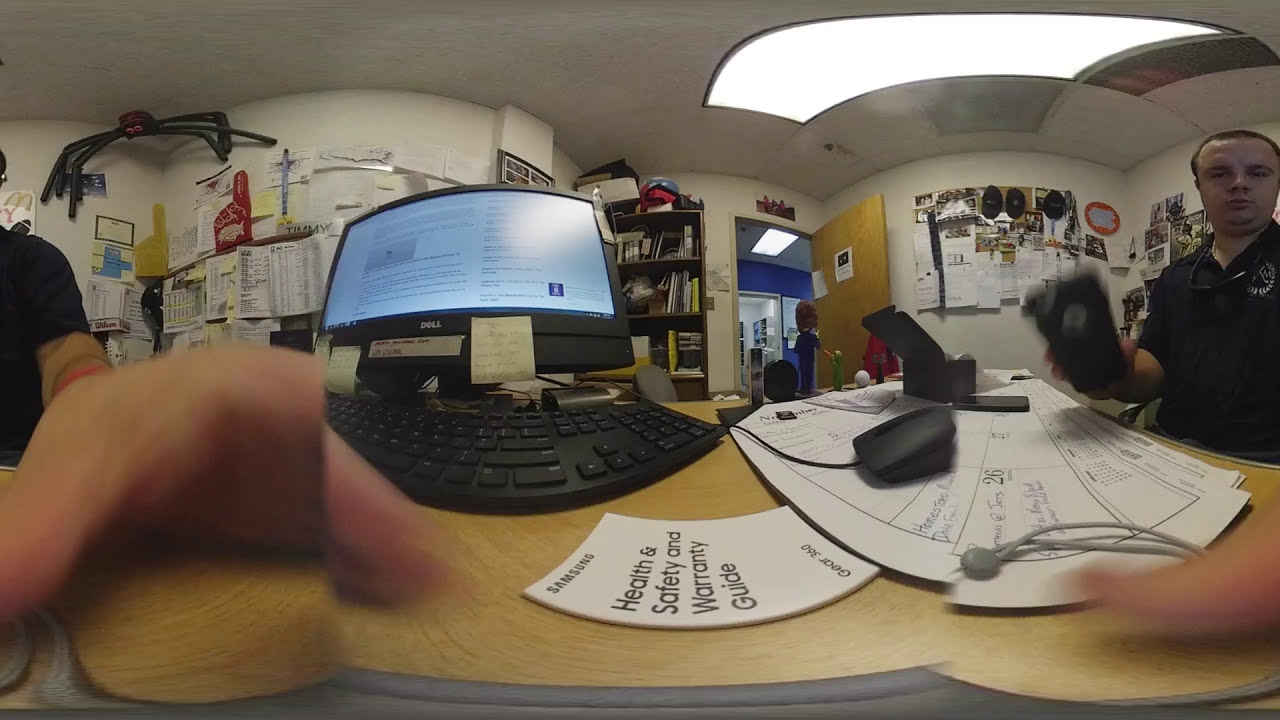This indoor photograph appears to be a composite created by stitching together three distinct images, resulting in a slightly curved and irregular visual effect. At the center of the image stands a workspace with a brown desk. On the desk, prominently placed, is a white booklet titled "Samsung Health and Safety Warranty Guide." A black Dell computer monitor and matching keyboard are positioned to the upper left of this booklet, with a large paper calendar on the far left of the desk.

In the middle background, we see a white wall adorned with shelves and an overhead light that subtly curves due to the stitching. To the left part of the image, there’s a man with Caucasian skin, dressed in a black polo shirt. He is seated behind the desk, holding a black camera or smartphone, seemingly engaged with the device. Further to the left, beyond the man, an open doorway leads to another section of the office space.

On the far right of the photo, the image shifts again to show the continuation of the composite. Here, only an outstretched arm in a black shirt reaching towards the camera is visible, with no face shown. In the upper left corner of the image, a spider decoration on the wall hints that the photograph might have been taken around Halloween. The combination of these elements—furniture, technology, human presence, and seasonal decoration—paints a vivid picture of a bustling office environment.